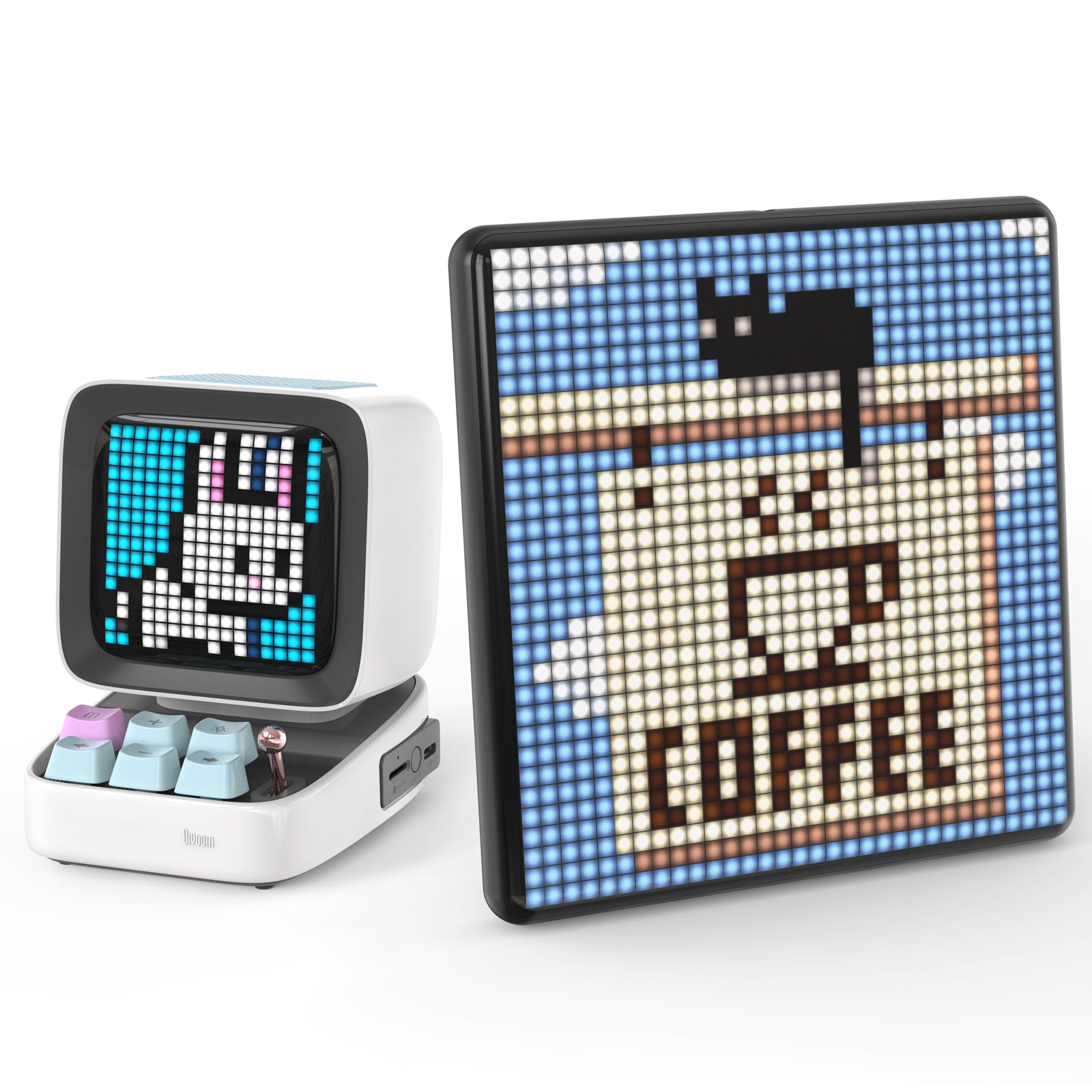The image depicts a detailed, pixelated art scene split across two distinct elements. On the left, a miniature, toy-like computer screen shows a pixel art of a rabbit with pink ears and a pink nose against a light blue background. This tiny, old-fashioned screen is accompanied by a six-button keypad and a lever, all designed to mimic vintage electronics and sized roughly like a cigarette pack, suggesting it is a playful, child-friendly gadget. 

To the right, occupying a larger portion of the image, is a bigger screen that showcases a complex mosaic picture. This scene features a black cat with cream-colored eyes and a long black tail draping over a wooden beam. The cat is perched atop a platform adorned with a prominently displayed coffee shop sign. The sign has dark brown markings depicting a coffee cup along with the word "COFFEE" in bold, capital letters, all set against a background of light blue with scattered white clouds. The coherent use of blue, black, brown, and white dots throughout the mosaic creates a visually appealing blend of digital and nostalgic aesthetics.